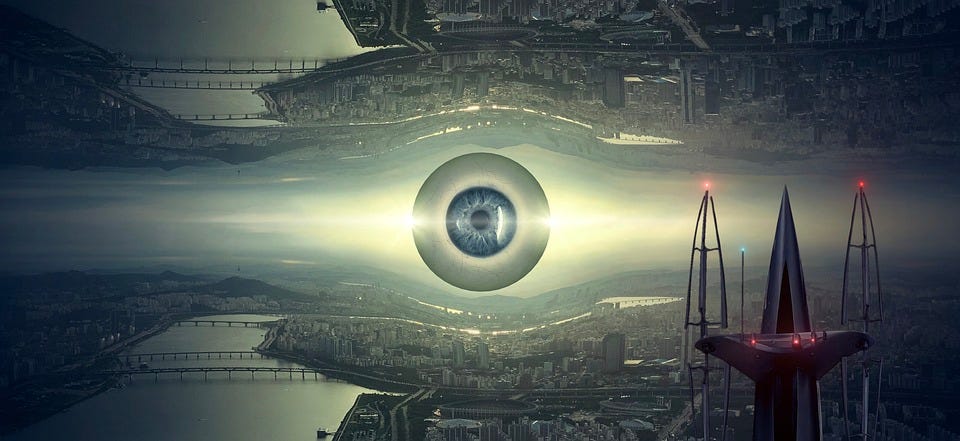In a surreal and dystopian style, this digital illustration features a central, realistic-looking blue eyeball, roughly the size of a planet. It hovers over a mirrored landscape, reflected symmetrically along the horizontal axis, creating an alternate dimension-like effect. Both the upper and lower halves of the scene reveal an extensive city skyline with a bridge leading to a sprawling metropolis. In the lower left corner, a distinctive structure equipped with red lights, akin to those on a radio tower, stands out. This structure also includes a helicopter landing pad or similar platform. To the right of the giant eye, an imposing tower with pointed pillars and additional red lights rises ominously, reminiscent of the eye of Sauron. The predominant colors in the image are various shades of gray and greenish gray, although the scene is punctuated by blues and reds, lending a vivid, surreal quality to the urban landscape. Shaded trees and distant mountains fill the background, enhancing the otherworldly atmosphere. Prominent light orbs shine from the back of the eye to the front of the image, elongating across the scene and further adding to the dystopian aesthetic.